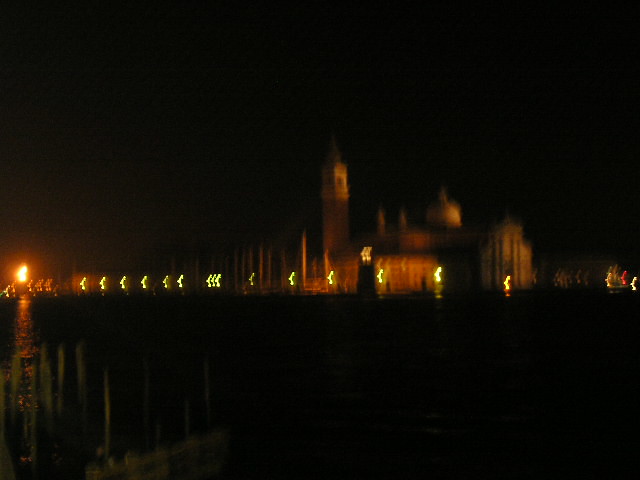The nighttime photo, characterized by significant blur, depicts a grand, castle-like structure majestically illuminated against a backdrop of complete darkness. The building in the background appears to be multi-storied and expansive, featuring a tall tower on the left, various smaller protruding towers in the middle, and a larger rounded tower on the right, giving it a vaguely European, possibly ecclesiastical feel. Street lamps cast an orange glow, highlighting the structure’s grandeur and providing the primary illumination in the image. These lights are visible along the horizon and appear to create reflections on what seems to be a body of water in the foreground, potentially a lake, with a dock faintly visible in the lower left corner. The image conveys a serene, almost eerie ambiance, with no people and an absence of natural light, encapsulating a silent, majestic night scene by the water.